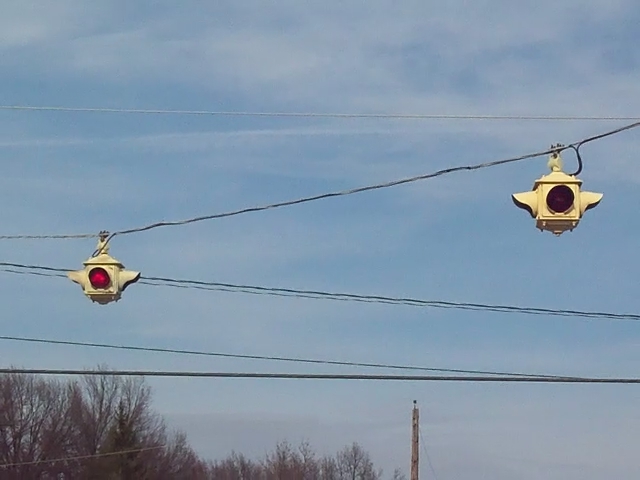The photograph captures a clear, medium-blue sky with wisps of clouds stretching across it. At the center of the image, two streetlights are suspended from a black cable in a four-way intersection setup. The streetlights, which are yellow, are the small, square kind with individual lights mounted on either side. The light on the left side of the image is showing red, signaling stop, while the other light is not illuminated. Below the streetlights, a series of electrical wires runs horizontally across the image. In the background, to the left, bare trees with dark brown trunks and branches provide a stark contrast against the vibrant blue sky. The landscape is minimalistic, leaning heavily on the interplay between urban and natural elements.